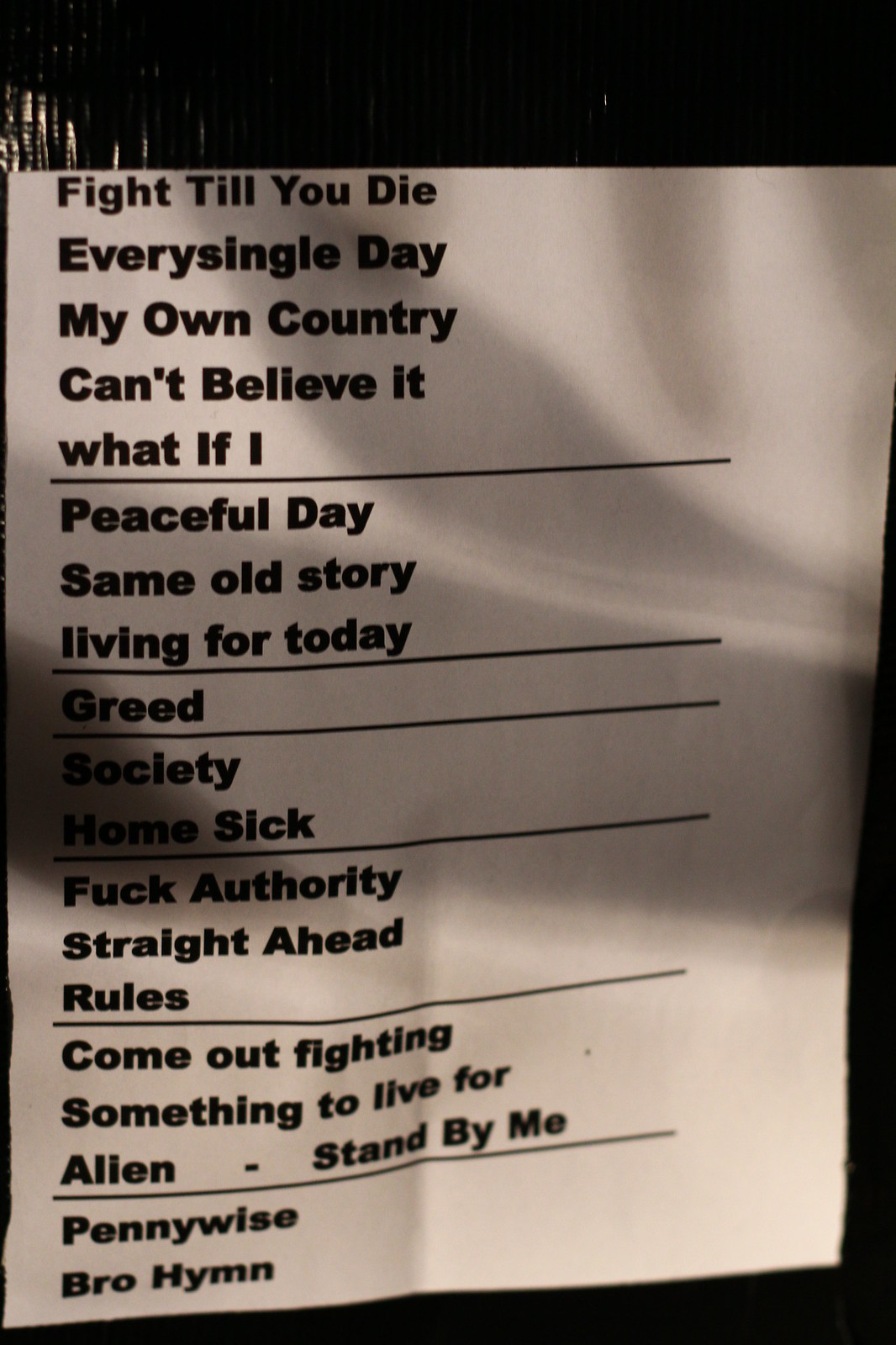The image displays a white piece of paper with black text, folded and partially shadowed at the center. It appears to be a setlist, possibly for a live music performance, featuring several bold-lined sections separating different song titles. Notable songs listed include "Fight Till You Die," "My Own Country," "Peaceful Day," "Same Old Story," "Greed," "Society," "Homesick," "Straight Ahead," "Come Out Fighting," "Something to Live For," and "Pennywise." The final song on the list is "Bro Hymn." The text layout is structured with various bold, dividing lines marking these sections. Additionally, a dark diagonal black bar crosses the paper, contributing to the shadows at the center. Furthermore, a leaf blade or similar object appears to overlay the midpoint from the center top to the right edge, adding to the composition's textured appearance. The only lowercase text is in "What if I" and "living for today," reflecting a deliberate stylistic choice.